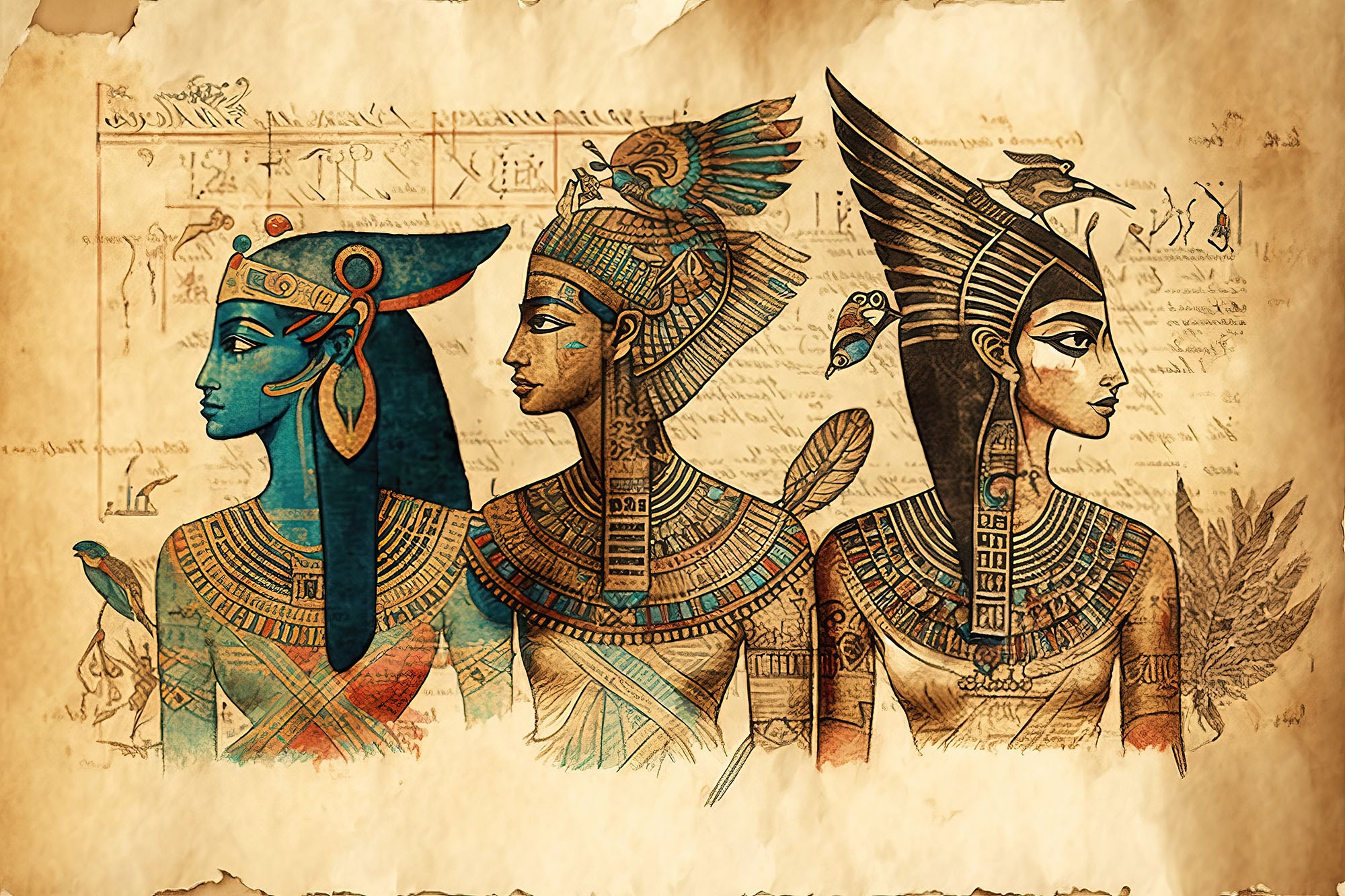The image is a detailed Egyptian-themed drawing featuring three figures against a background designed to resemble weathered, crumbling papyrus paper. This backdrop is tan and brown in color, filled with faded, illegible text and symbols that mimic ancient hieroglyphics. The top and bottom edges of the paper are torn or chewed, enhancing its aged appearance.

In the foreground, three figures are depicted from the stomach upwards. On the left is a woman with striking blue skin, adorned with a gold-colored shoulder piece and a red robe. She wears a curved black hat with a gold brim. The central figure is a man wrapped mostly in bandages, with gold-colored skin and a richly decorated gold headdress topped with a peacock. He also sports a gold-colored neck piece. To the right is another woman with light-colored skin, wearing a sweeping black and white hat. All three figures exude an aura of historical Egyptian grandeur, brought to life with vibrant headdresses and accessories.